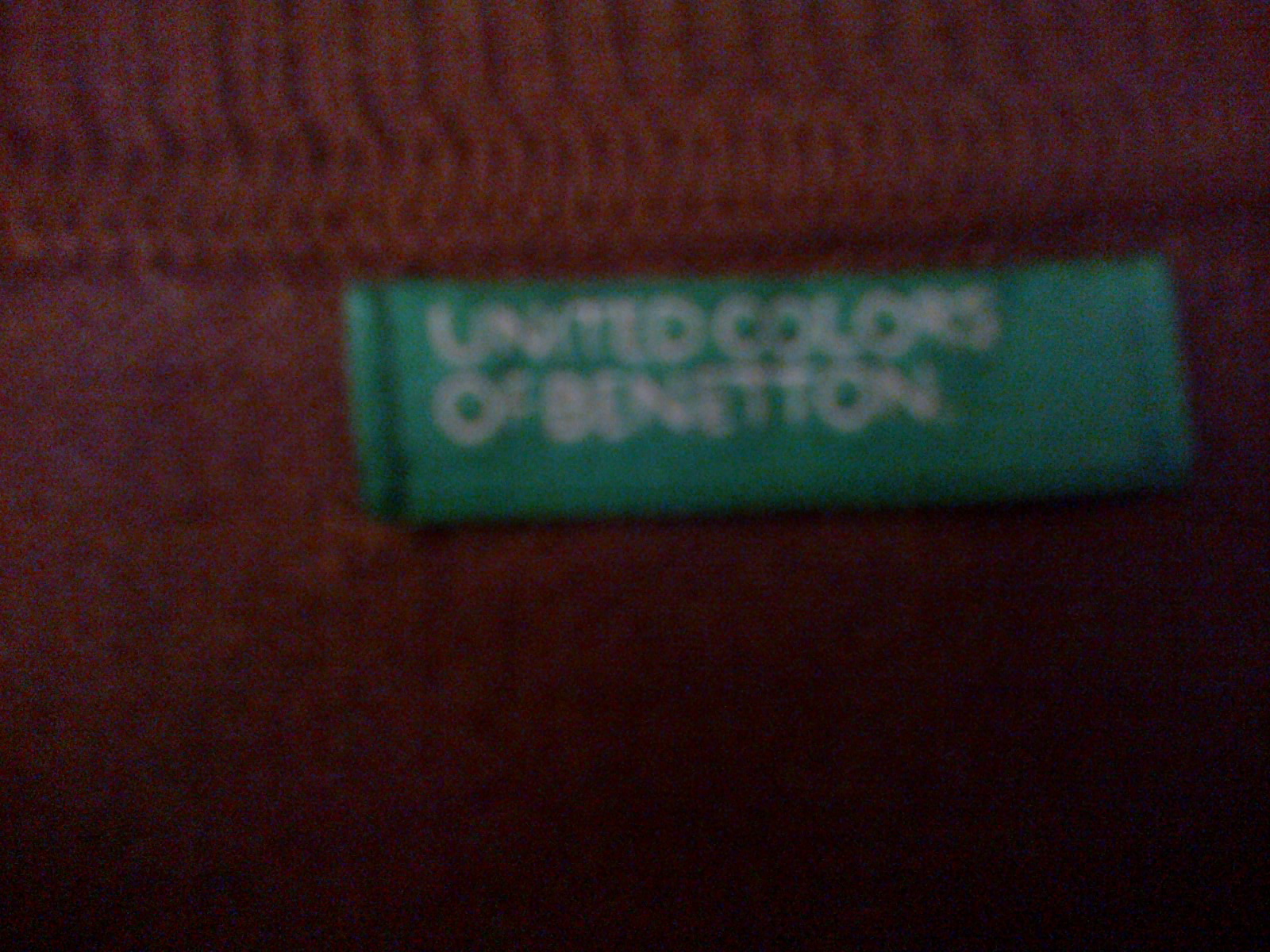This is a very blurry close-up photograph focusing on a clothing label sewn into a garment. Due to the tight framing, the actual item of clothing is indiscernible, but it features a dark red, rust-colored fabric. The label itself is small and green, with white text that reads "United Colors of Benetton." It appears to be stitched in right at a seam. Above the seam, the material has a ribbed pattern, suggesting that the fabric might be the cuff of a sleeve or the hem of a stretchy, ribbed shirt.